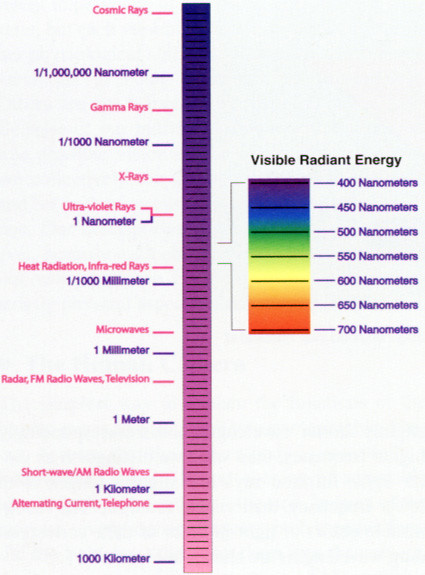The image is a detailed rectangular chart with a white background, primarily split into two sections. The left side features a long vertical gradient bar starting with dark purple at the top and transitioning to light pink at the bottom. This gradient visually represents the electromagnetic spectrum from high-energy cosmic rays at the top to low-energy alternating current at the bottom. Specific terms like gamma rays, X-rays, ultraviolet rays, heat radiation, infrared rays, microwaves, radar, FM radio waves, television, shortwave AM radio waves, and alternating current telephone are labeled alongside respective wavelengths, ranging from one one-millionth of a nanometer to 1,000 kilometers.

On the right side, there is a stack of rectangles representing visible radiant energy, each rectangle divided by a black line and color-coded from purple to blue to green, yellow, orange, and ending at red. These rectangles are labeled with corresponding wavelength measurements from 400 nanometers (purple) to 700 nanometers (red) at 50-nanometer intervals, showcasing the visible spectrum. This section provides a clear guide to the visible light spectrum in nanometers.

Overall, the chart comprehensively displays the entire electromagnetic spectrum, grouping various types of radiation and waves based on their wavelength and color, effectively illustrating the range and classification of different forms of energy.